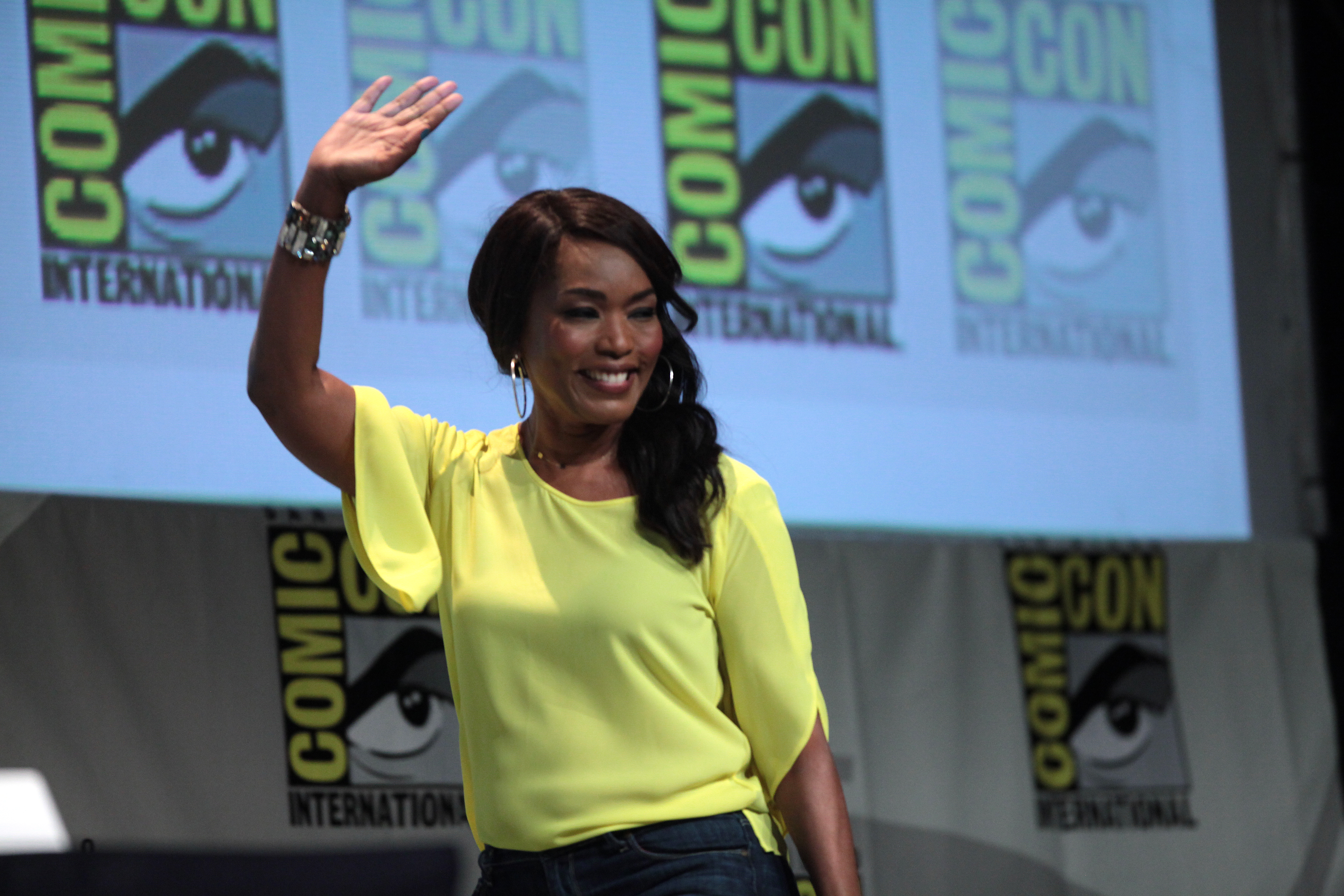The image depicts an African-American woman who closely resembles Angela Bassett, although she is not her. She's standing on a stage, waving with her right hand adorned with a chunky silver bracelet. She is wearing a neon yellowish-green top made from a light, chiffon-like material with flowy sleeves, paired with dark blue denim jeans that are visible up to just below her waistline. Her ensemble is complemented by large silver hoop earrings and maroon lipstick, and her dark, wavy hair is stylishly swept to one side. The background features a banner with the Comic-Con International logo, which consists of four square panels each displaying a stylized eye graphic. The text "Comic" runs vertically up the left side of the squares, and "Con" runs horizontally across the top, both in neon green font, with "International" written along the bottom of the rectangles.